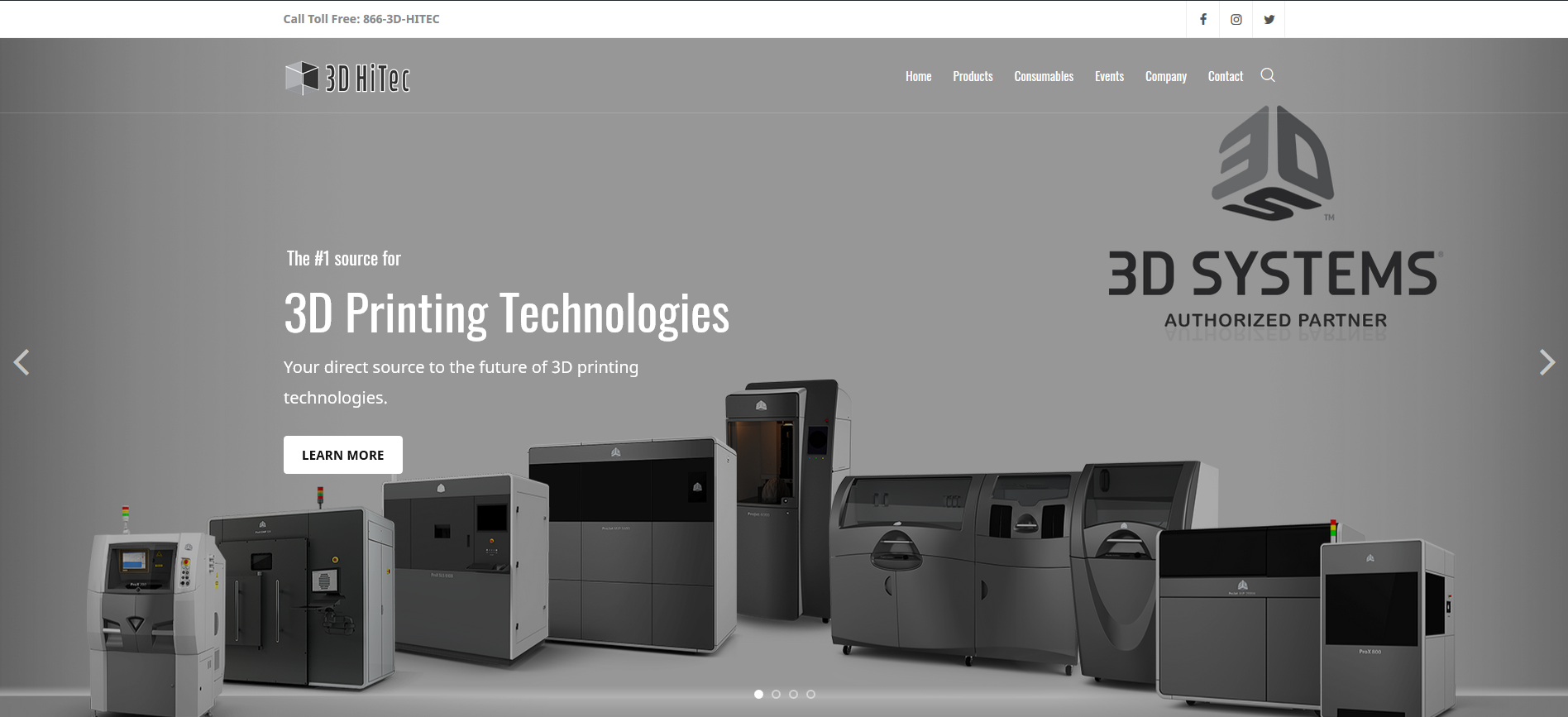The homepage of the 3D HiTECH website showcases their specialization as an authorized partner of 3D Systems. The gray background of the site prominently features the phrase "Your Number One Source for 3D Printing Technologies," emphasizing their position as a key provider in the future of 3D printing innovations. The header includes navigation links such as Home, Products, a section with smaller, unreadable words, Company, and Contact, along with a magnifying glass icon for search functionality.

Dominating the main section of the page is an image of several industrial-grade 3D printers. These machines are large and robust, resembling appliances more than consumer-grade 3D printers. The image is in grayscale, giving the printers a solid gray appearance which might be attributed more to the photography than their actual colors.

Additional elements on the page include a white "Learn More" button and social media icons for Facebook, Instagram, and Twitter. Also prominently displayed is a toll-free contact number. Users can navigate the site further by scrolling to the right, as suggested by the presence of navigation links.